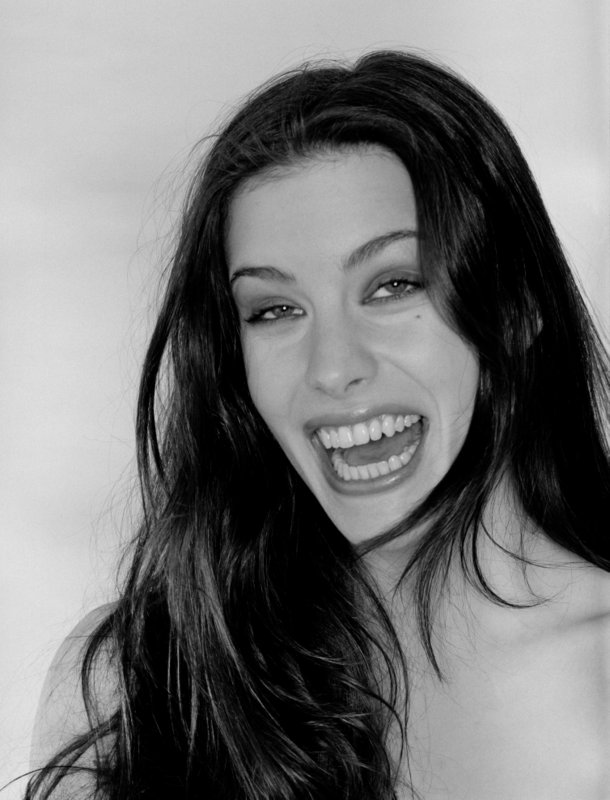This black and white photograph captures actress Liv Tyler, daughter of Steven Tyler of Aerosmith, from just above the chest up. She has long, flowing dark hair that extends past her shoulders, partially obscuring her chest area. Liv is depicted with her mouth wide open, revealing straight rows of top and bottom teeth. Her eyes are half-closed, giving her a slightly dazed yet happy expression, possibly mid-laugh or mid-cough. She sports distinct, curvy eyebrows and a noticeable mole under her right eye. The background appears grayish, but this could be due to the black and white nature of the photo. It's a candid and expressive portrait that captures a spontaneous moment.